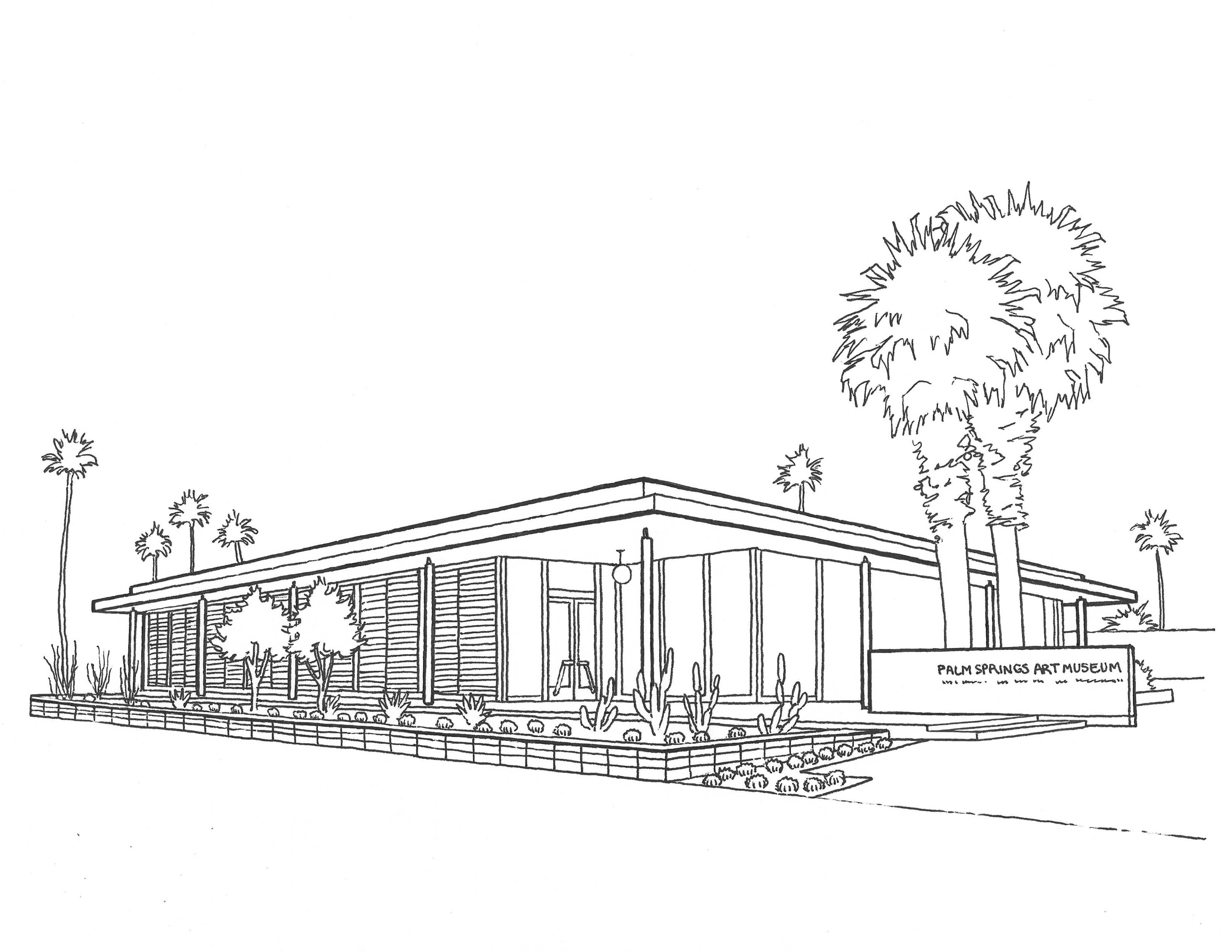The black and white line drawing depicts the Palm Springs Art Museum, a modernist, mid-century building characterized by its low profile and flat roof. Prominently featured is a sign in front that reads "Palm Springs Art Museum," confirming its Palm Springs, California, setting. The building is surrounded by an array of palm trees—two of which are massive and stand directly behind the sign, additional palms are situated behind the building and to the left. A distinctive xeriscape garden flanks the left side and partially the front, hosting a variety of cacti, yucca trees, and small shrubby plants, as well as a thin palm tree.

The building itself appears to be constructed of wooden paneling and is a single-story structure. The front entrance, centrally located, features a couple of low cement steps leading up to a glass door, alongside which hangs a single outdoor pendant light. The overall composition of the drawing marries architectural precision with the charm of a New Yorker cartoon style, capturing the simplicity and quaintness of the museum’s design.